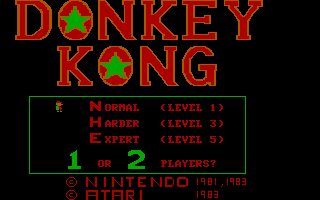The image is a screenshot of the title screen from the video game Donkey Kong on the Atari 2600. The entire background is black, with a prominent red Donkey Kong logo at the top, each 'O' replacing the circle with a green star. Below the logo, there is a black rectangle outlined in green, containing multiple lines of red text indicating difficulty levels and modes. The selectable options include Normal (Level 1), Harder (Level 3), and Expert (Level 5). Player selection is also available, with the options '1' and '2', written in green, visually standing out against the surrounding red text 'Or' and 'Players?'. Outside the rectangle, additional red text denotes the copyrights: 'Nintendo, 1981-1983' and 'Atari, 1983'. An orange outline accompanies the Donkey Kong logo, adding a classic touch, and to the left of the Normal selection, there is a small sprite of Mario (known as Jumpman in this game), indicating the current selection.